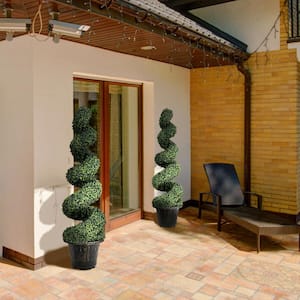This is a detailed, AI-generated photograph (or possibly a photorealistic illustration) depicting the back patio of a house on a sunny day. The focus is on a glass sliding door with brown framing, leading to the entrance of the home. This door is flanked by two identical, topiary-style plants, each spiraling upward and potted in black containers. The white wall of the house contrasts with a yellow brick section to the side, forming part of the patio's backdrop. The patio itself features brick pavers, with red and brown cobblestones adding texture to the walkway. To the right of the entrance, there is a black chaise lounge positioned for optimal sunbathing. Additionally, the patio is illuminated by Christmas lights strung across the area, hinting at a winter season. Two security cameras are mounted under a brown roof overhang, which also casts shadows from the twisted topiaries. The overall impression is one of a well-maintained and secure outdoor space, combining functional and decorative elements harmoniously.